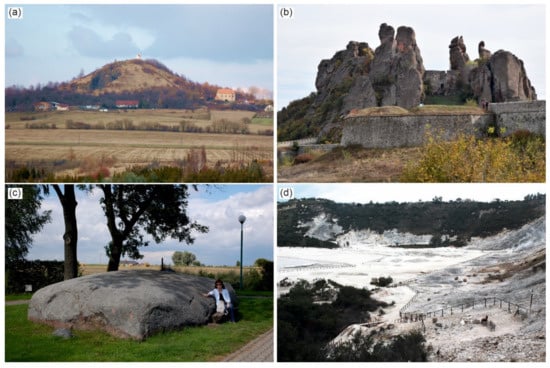This image is divided into four equal sections, each featuring a different photograph labeled A, B, C, and D. In the top left section (A), there's a scenic view of a mountain range under a bright blue sky with some scattered blue clouds. In the foreground, there's a mixture of brown grass with patches of green, a few distant houses, and trees lining the landscape. The top right section (B) presents a close-up of a rocky cliff with black and gray stones. The sky, still blue, contrasts with the dark rocks and surrounding greenery, including trees. The bottom left section (C) features a large rock formation surrounded by trees, with a person kneeling beside it, touching the rock. This image is also taken during the day under a blue sky. Lastly, the bottom right section (D) displays a snowy landscape with a man-made hand railing descending what appears to be a mountainside or cliff. The entire scene is blanketed in snow, except for some distant trees that are relatively less snow-covered. The overall color palette of these natural outdoor scenes includes brown, white, black, light green, dark green, gray, blue, tan, and beige, with all photos captured in daylight.